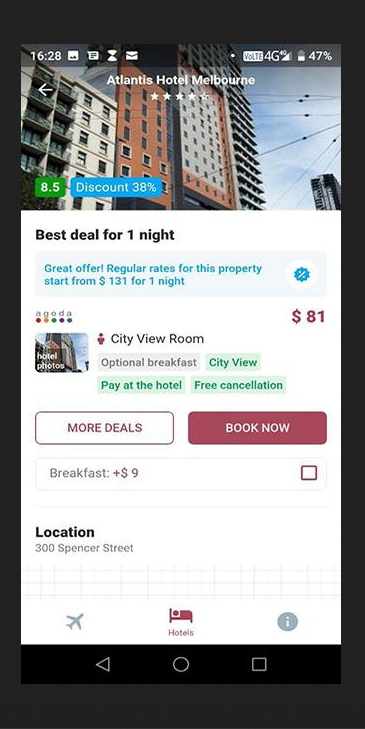A close-up of a tablet screen displaying a hotel booking page for the "Atlanta Hotel Melbourne" at 1628. The screen’s top section reveals device status indicators: "Volt E" icon, 4G signal, and battery level at 47%. The background is black.

The tablet’s top third showcases a cityscape, possibly of New York City, featuring a mix of high-rise buildings—including an orange-brick structure with balconies. Overlaid on this image, the words "Atlanta Hotel Melbourne" appear in bold, followed by four white stars and a transparent star, an 8.5 rating in a green box, and a "38% discount" notification in white font inside a blue box.

Beneath the cityscape, a white box with "Best deal for one night" in black font is displayed. Below it, a note mentions the great offer: regular rates start from $131 per night, highlighted in blue font.

The tablet screen is divided into three sections. The left section includes a clickable thumbnail for hotel photos and states "City View Rooms" with a small icon of a person. The price $81 is displayed in brown font at the top right of this section. Below, features such as "Optional breakfast," "City View," "Pay at the hotel," and "Free cancellation" are listed. The "Optional breakfast" is in a grey box with dark grey font, while the other features are in green boxes with green font.

Two prominent buttons are found below: an orange-background button labeled "More deals" and a reddish button labeled "Book now."

Further down, there is a checkbox option for "Breakfast plus $9". The hotel location is listed as "300 Spencer Street" in black font.

The bottom of the screen features three icons: an airplane, a hotel bed with a person, and an information (i) symbol. At the very bottom, there are controls resembling a play button, a pause/halt button, and a square button, likely for media control.